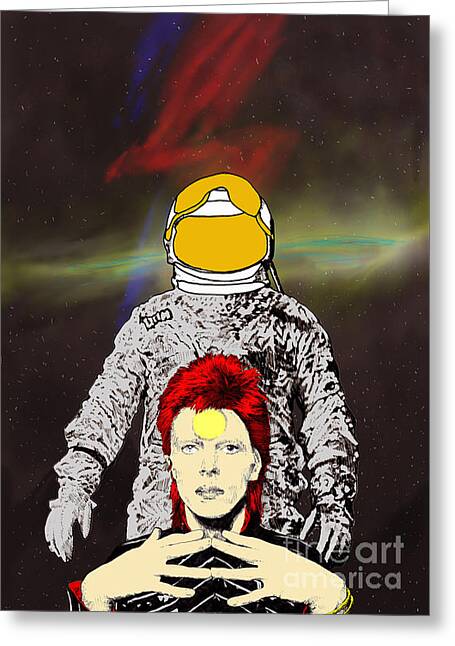The image is an artistic, semi-realistic drawing featuring David Bowie and an astronaut set against a cosmic background. David Bowie, portrayed with bright red hair and a yellow circle on his forehead, is positioned at the bottom front of the image, facing forward with his fingertips touching just below his chin. He is dressed in black, and from his chest down, the details are cut off by the bottom of the frame. Behind him stands an astronaut in a white-gray crinkly suit with a cartoonish white and yellow helmet. The backdrop is a mesmerizing outer space scene, predominantly black with scattered stars and a multicolored galaxy. Adding dynamic visual elements, there is a glowing green and yellow horizontal stripe and a red zigzag pattern overlapping a blue stripe. The image, credited to Fine Art America with a watermark in the bottom right corner, is a striking blend of vivid colors and imaginative design, reflecting the artist's admiration for David Bowie.